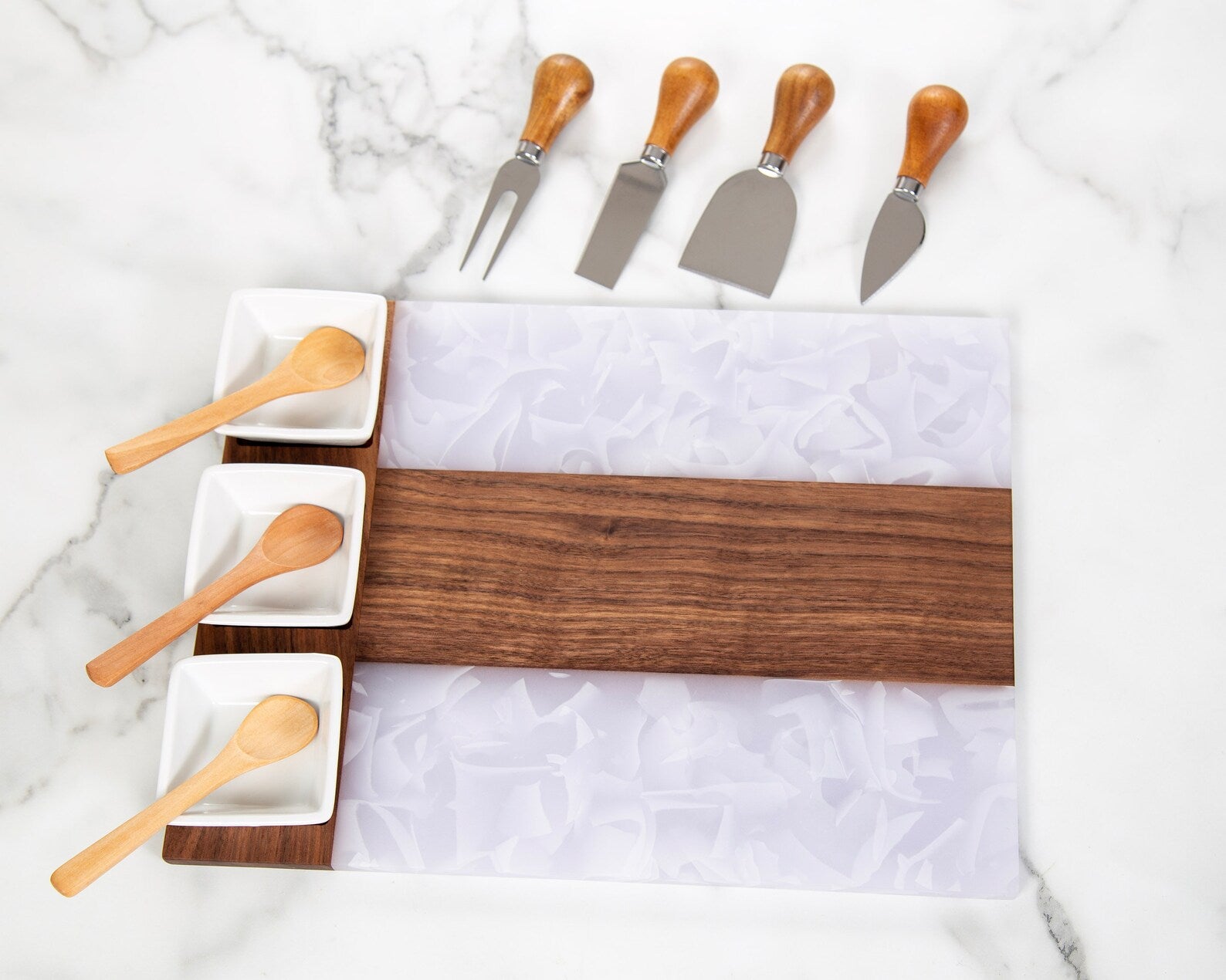The image depicts a bright, indoor kitchen setting featuring a primarily white, marbled countertop veined with gray streaks. Resting on this countertop is a distinctive, rectangular serving tray or cutting board. The tray is segmented, with its right-hand side divided into three horizontal sections: the top and bottom sections are white plastic, while the center section is a brown wooden plank. On the left side of the tray is another wooden slat holding three small, white square dishes, each accompanied by a wooden spoon positioned diagonally with their handles pointing towards the bottom left. Above this tray, four kitchen utensils are neatly arranged. These utensils, which include a cake server, a wide spatula, a narrow spatula, and a two-pronged fork, feature wooden handles and metallic ends, adding a touch of rustic elegance to the modern kitchen scene.